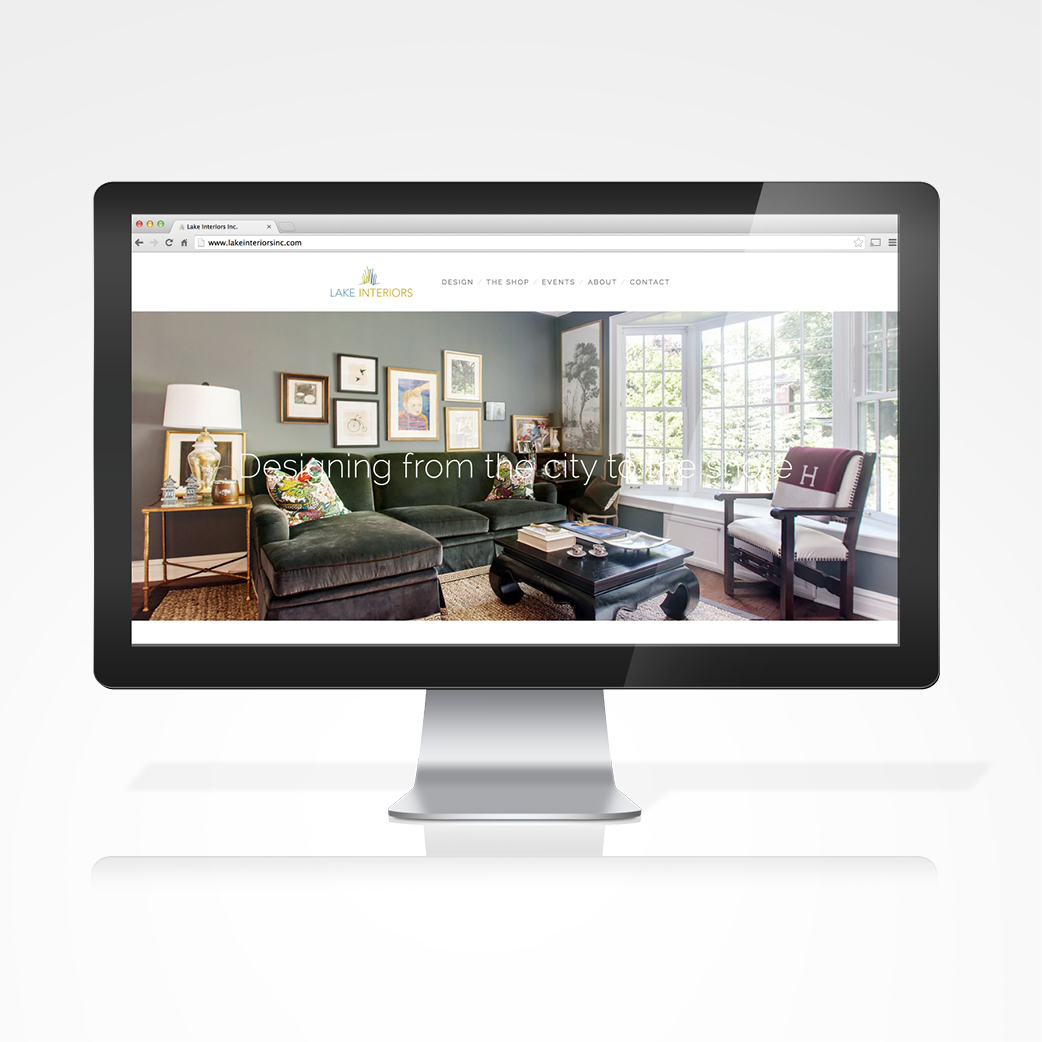This screenshot, presumably from a website displayed on a desktop PC, highlights an advertisement or webpage for an interior decorating or furniture company called "Lake Interiors." The top of the page features a navigation bar on a white background, allowing users to explore various products and services offered by the company.

Dominating the main portion of the page is an image showcasing a stylishly designed living space. The centerpiece is a black sectional couch, accompanied by the text "Designing from the City" in white lettering. The couch, though modest in size, looks inviting with two large pillows adding to its comfort appeal.

In front of the sectional couch, a black wooden coffee table holds several items, including a book and some coffee cups, indicating a lived-in, cozy environment. Adjacent to the coffee table, there is a polished wooden chair with brown and white cushions, positioned beside a large, brightly lit window which floods the room with natural light.

Behind the sectional couch, six art pieces adorn the wall, adding a touch of sophistication. To the right, a much larger painting depicting a tree stands out, contributing to the room's artistic ambiance. 

Next to the couch, a smaller side table supports an elaborate lamp and additional decor items, enhancing the room's aesthetic appeal. The floor features a brown rug over wooden planks, further adding to the room's warm and inviting feel.

Overall, this well-lit, tastefully decorated room exemplifies the design expertise of "Lake Interiors," offering a glimpse into the comfortable and stylish living spaces they can create for their clients.